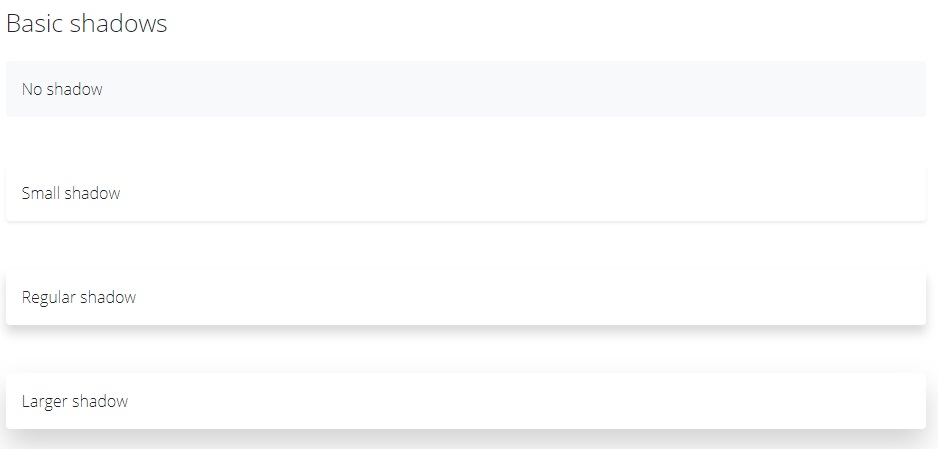A monochromatic diagram displaying various types of shadows on a white background. At the top, the title "Basic Shadows" is prominently displayed. Below this heading, four sections are labeled as "No Shadow," "Small Shadow," "Regular Shadow," and "Larger Shadow," respectively. Each section is devoid of photographic or illustrative elements, focusing purely on textual descriptions without any color. The image is devoid of people, animals, birds, fish, insects, plants, flowers, trees, buildings, or any man-made structures. Additionally, there are no natural landscapes such as mountains, or any transportation vehicles like automobiles, airplanes, helicopters, boats, or motorcycles. The image is strictly an informative text depiction of shadow sizes in various scenarios.